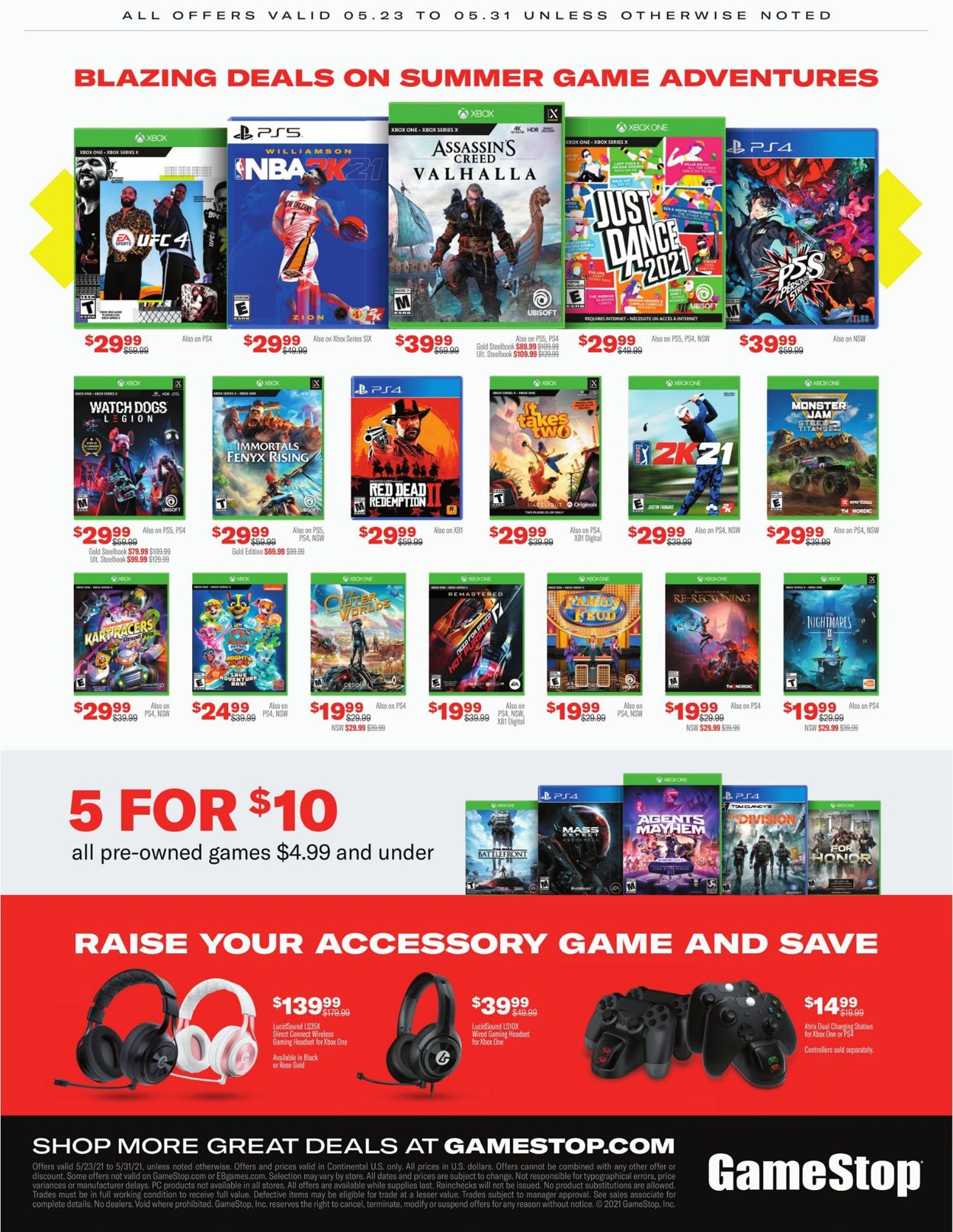The image depicts a GameStop sale advertisement showcasing various deals on gaming accessories and games. At the bottom right corner, inside a black bar, the GameStop logo is prominently displayed with a message encouraging shoppers to find more great deals at GameStop.com, though the finer print is too small to read. Just above this, a red bar highlights a promotion: "Raise Your Accessory Game and Save," offering three types of accessories. There’s a brand of headphones priced at $139.99, another brand at $39.99, and controllers available for $14.99. Moving upwards, a gray bar features a "5 for $10" sale for all pre-owned games priced at $4.99 and under, with five game covers shown as examples—three for Xbox and two for PlayStation. 

Dominating the upper half of the page is a vibrant call to action: "Blazing Deals on Summer Game Adventures." This section is organized into three rows. The first row displays five games priced between $29.99 and $39.99. Below, the second row offers five games all uniformly priced at $29.99. The final row lists seven game covers with prices ranging from $19.99 to $29.99. All featured games are available for either Xbox or PlayStation platforms.